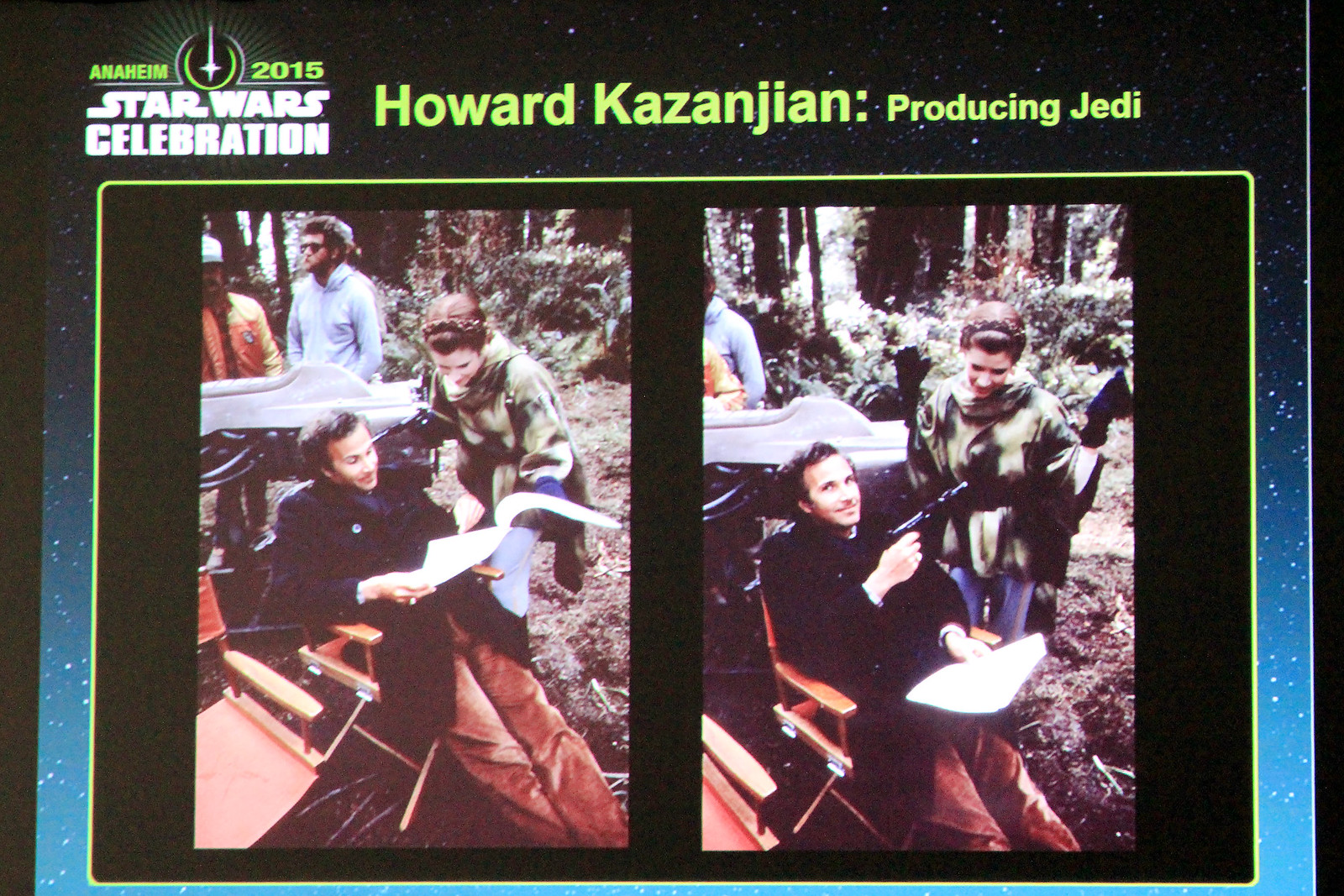The image appears to be a photograph of a projected screen showing two side-by-side panels, each framed within a green border and surrounded by a black space with a subtle starry background. At the very top, bold text reads "Anaheim 2015" with a small star logo, indicating the "Star Wars Celebration." Below this, in green text, it says "Howard Kazanjian Producing Jedi." 

The two panels depict behind-the-scenes moments from "Return of the Jedi." In both images, producer Howard Kazanjian is seated in a director's chair, wearing a long-sleeve blue shirt, jacket, and brown pants with his legs outstretched. Beside him, Carrie Fisher, dressed as Princess Leia in her iconic camouflage outfit and braids, is engaged in reviewing the script with Kazanjian. One photo captures Kazanjian focused on the script while Fisher looks on, and the other shows him smiling directly at the camera while holding Princess Leia's blaster, as Fisher laughs. The scene is set against a forest backdrop with some crew members in the background, enhancing the authenticity of this behind-the-scenes glimpse.